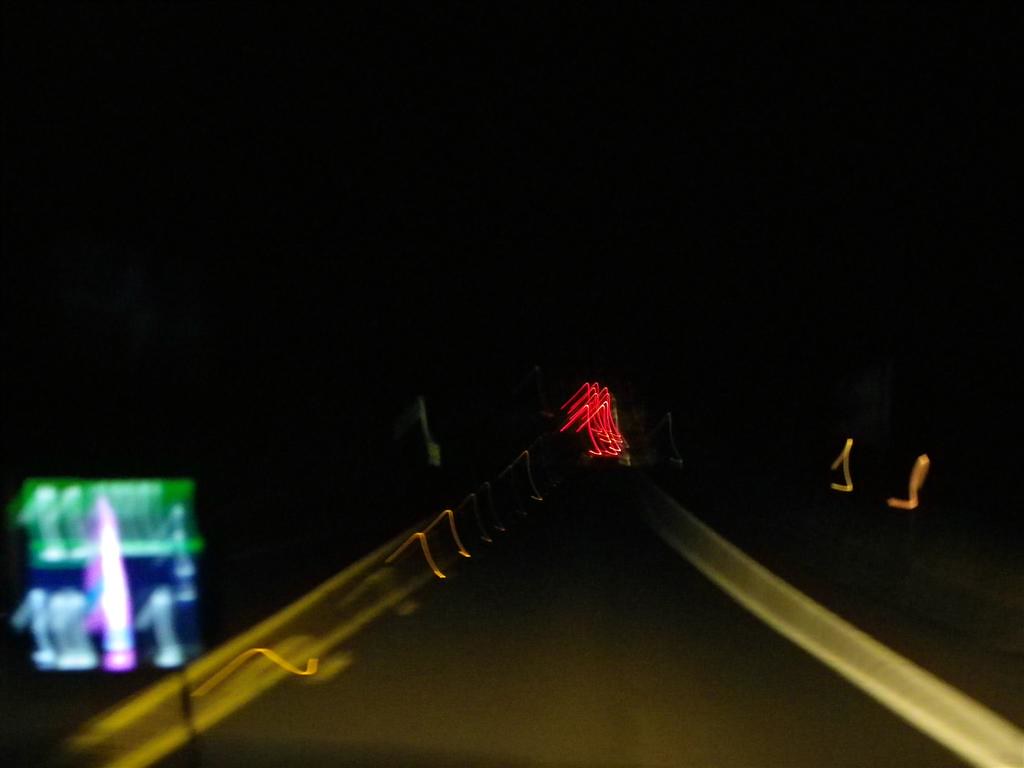A nighttime photograph appears to have been taken from a moving vehicle or by someone running on a road. The majority of the image is cloaked in darkness, but yellow street lines are visible on both the left and right sides, converging towards the center in the background. In the left foreground, there are two signs, likely a single sign captured with a motion-induced ghost image. The sign displays "11-1" with a dark blue background on the bottom and a green top, possibly a standard street sign. Reflectors are scattered throughout the scene, their lines of light stretching across the image, intermingled with streaks from the brake lights of a distant car, emphasizing the motion of the photograph.